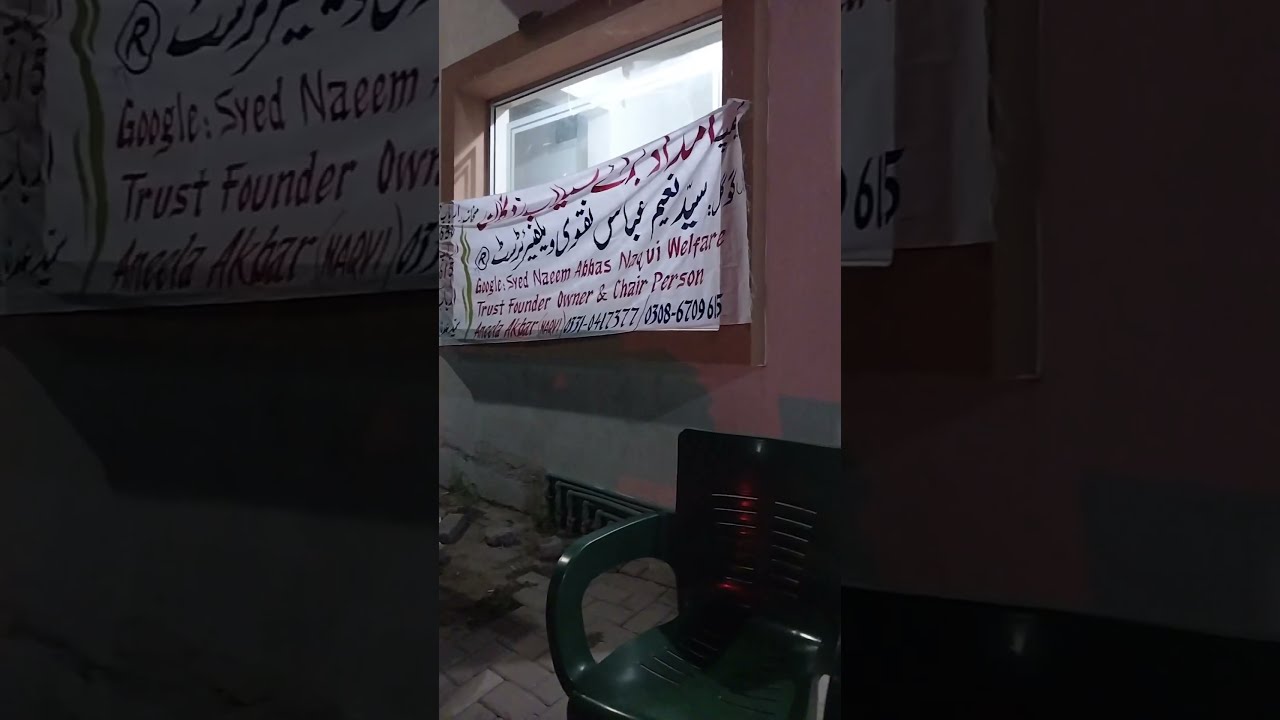The image showcases a somewhat disorganized and dilapidated room with old construction elements. In the center of the photo is a wooden-framed rectangular window, with bright white light streaming through. A fabric banner hangs halfway up the window, partially blocking the light. The banner features text in a foreign script, likely Arabic, and prominently displays the red letters "Google Syed Naeem", followed by "Trust Founder, Owner and Chairperson" in black text and some contact information. The sections on the left and right of the image, tinted and zoomed in, focus on this text.

In the bottom right corner of the photo, there's a green plastic chair with slits cut out of its back, reflecting some of the light. The floor beneath the window is tiled, but many of the tiles are broken. There's a vent at the bottom of the wall with a crack extending from it towards the left. The walls show signs of aging, with shadows giving them a pinkish hue, and the overall appearance of the room suggests it is in a somewhat run-down, abandoned state.